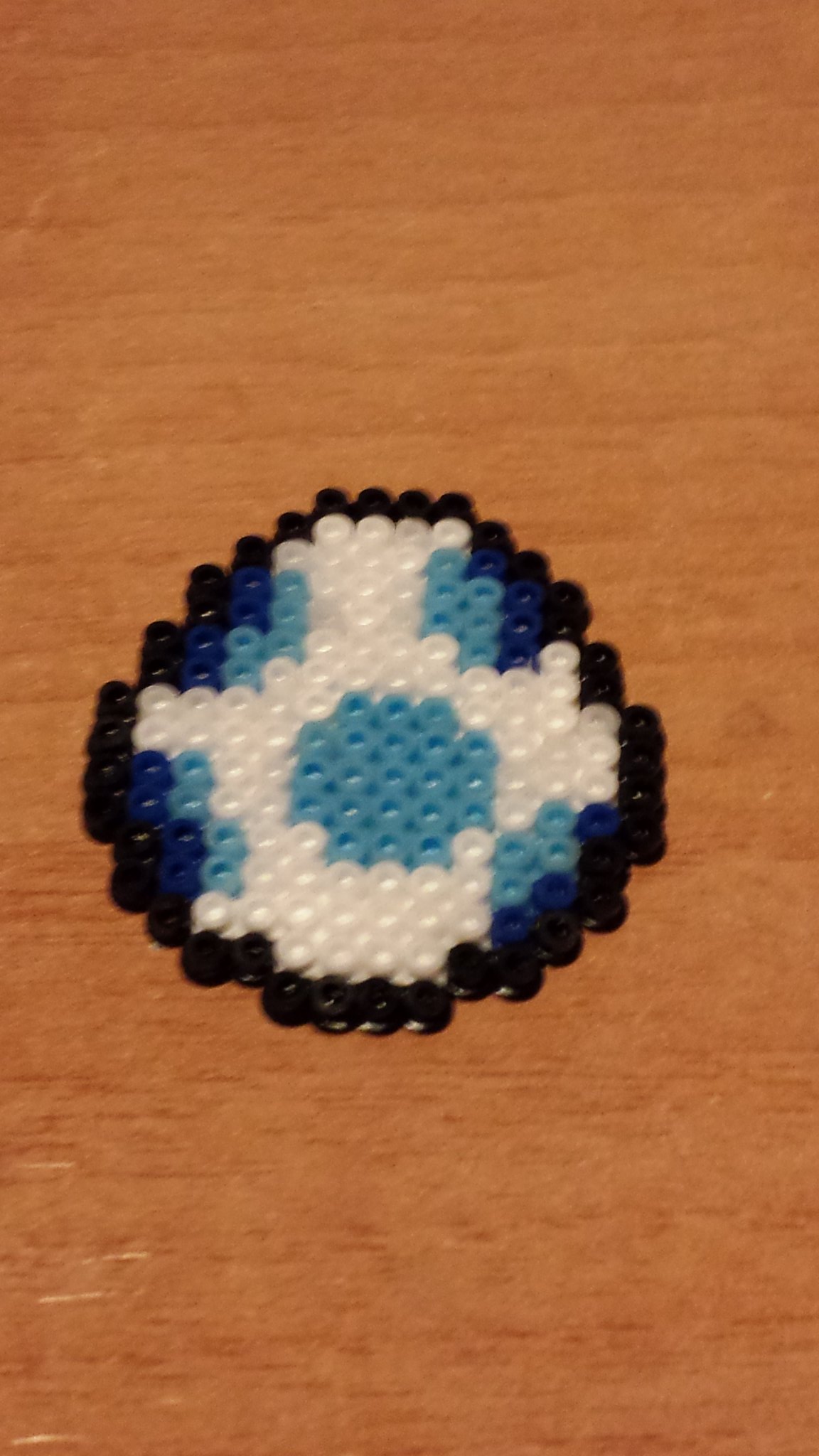The image depicts a small, abstract piece of art crafted from around 150 cylindrical Perler beads, measuring approximately 2.5 inches tall and 3 inches wide. This art lies flat on a brown wooden table and appears somewhat blurry. The creation features a central round light blue circle, encircled by white beads. Surrounding the white field are four splotches of light blue beads, each bordered by dark blue beads. The entire piece is edged with a single row of black beads, providing a distinct outline. The pattern does not represent any specific, identifiable object.